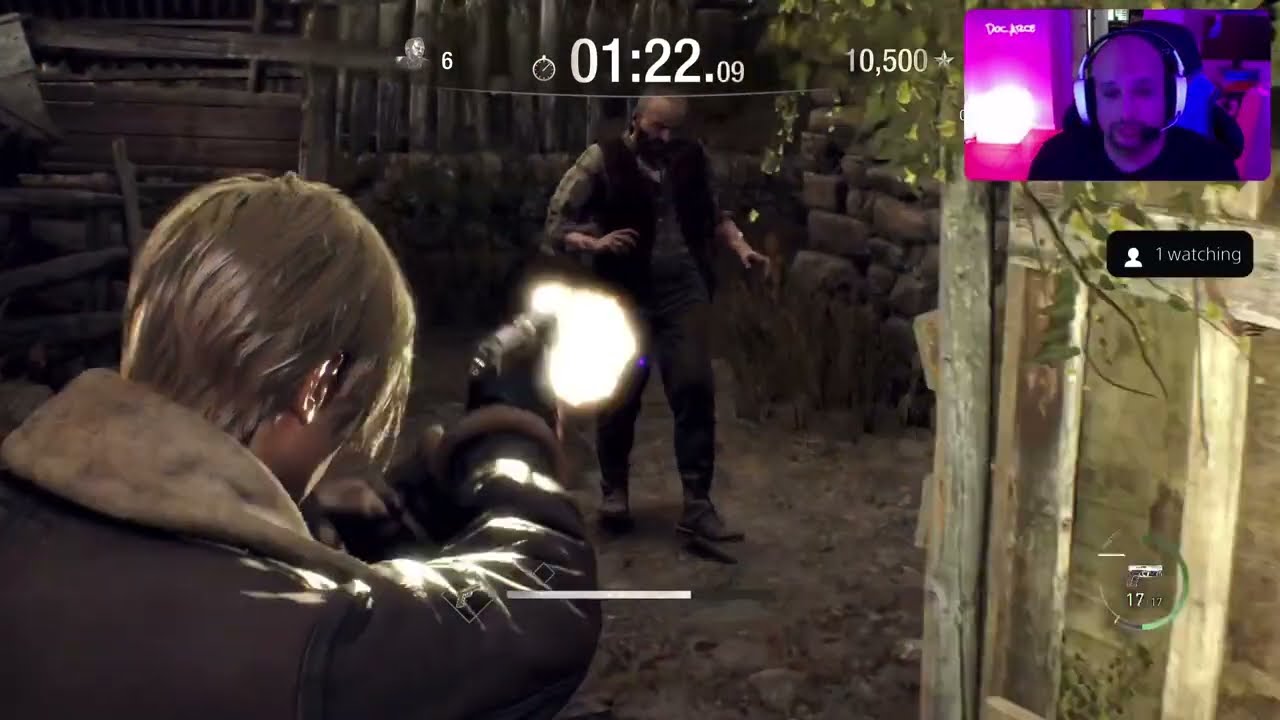This is a detailed screen grab from a recent Resident Evil video game, showcasing a third-person shooter perspective. The main game character, located in the lower left corner, is viewed over his shoulder. He sports a black jacket with a furry collar and has medium-length blonde hair, as he fires his gun at a zombie situated centrally in the image. The environment is dark, featuring a rough stone floor with a wood barn and rock walls in the background. Additional wooden logs are also visible. A scoreboard at the top of the image indicates a timestamp of 1-22-09 and a score of 10,500 with a star icon beside it. In the upper right, there's an inset of the live streamer playing the game. The streamer, who appears bald with a beard and mustache, is wearing white headphones and is illuminated by magenta, purple, and blue lighting. A white light is also visible to his left. Below his thumbnail, a black rectangle shows that there is "one watching" the stream. The overall color palette includes tan, brown, black, white, gray, pink, purple, and magenta.